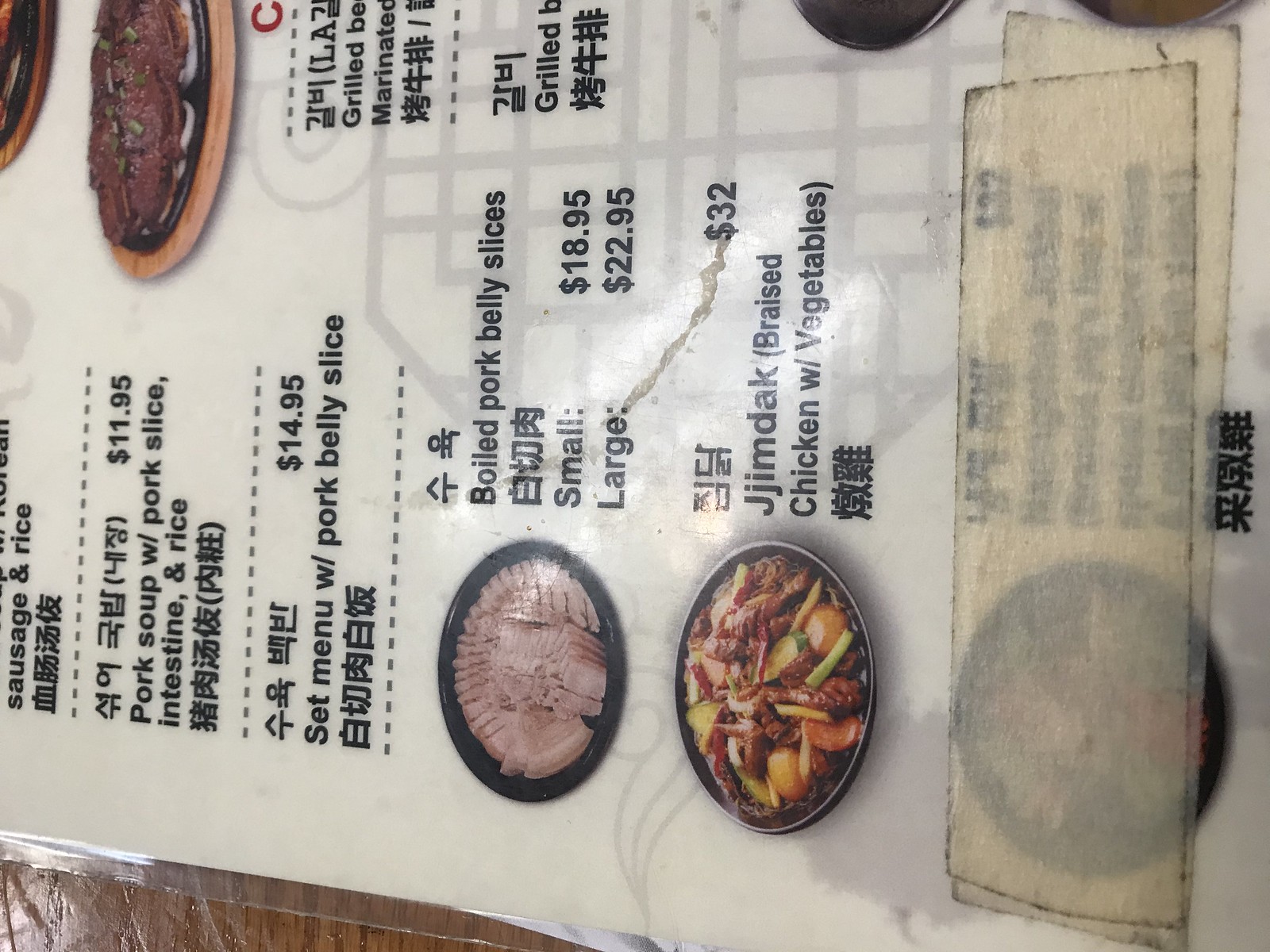On a rustic brown table, there lies a menu written in a foreign language, possibly Chinese, with some sections in English. The white menu with black print is adorned with vibrant pictures of delectable dishes, providing a visual feast for the eyes. 

Highlighted offerings include:
- Pork Soup with Pork Slices and Intestine, priced at $11.95.
- Set Menu Pork Belly Slice for $14.95.
- Boiled Pork Belly Slices, available in small for $18.95 and large for $22.95.
- Jimdak Braised Chicken with Vegetables for $32.00.

One section of the menu appears obscured, adding an air of mystery. The photographs feature an array of dishes served on elegant black plates. The pork belly slices, tinged with a delicate pink, hint at their succulence. The Jimdak braised chicken dish showcases tender slices of chicken paired with vegetables such as potatoes and zucchini. The spread is a tantalizing preview of the culinary delights awaiting patrons.